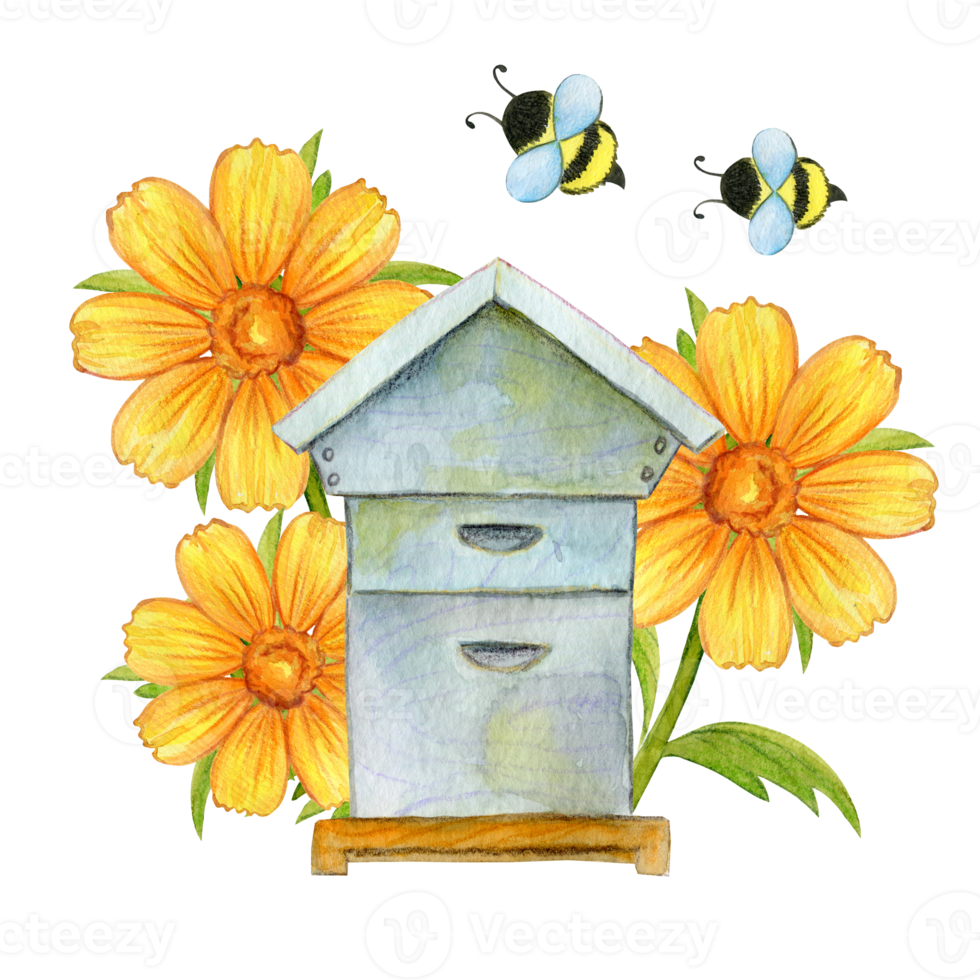This is a slightly cartoonish, hand-drawn and possibly hand-painted image of a man-made beehive typically used by backyard beekeepers to harvest honey. The beehive is depicted in shades of gray and green, resting on a brown platform. Behind the beehive, there are three large, sunflower-like flowers with round centers and multiple petals. The flowers are primarily orange with greenery visible behind them. Above and to the right of the beehive, two black-and-yellow bumblebees are shown flying—one straight and the other diagonally. The bees are viewed from the back, highlighting their fuzzy bodies and antennae. The majority of the background is white, making the central elements stand out. This charming and simple print could be a fitting decoration in a boutique shop or craft store like Hobby Lobby.